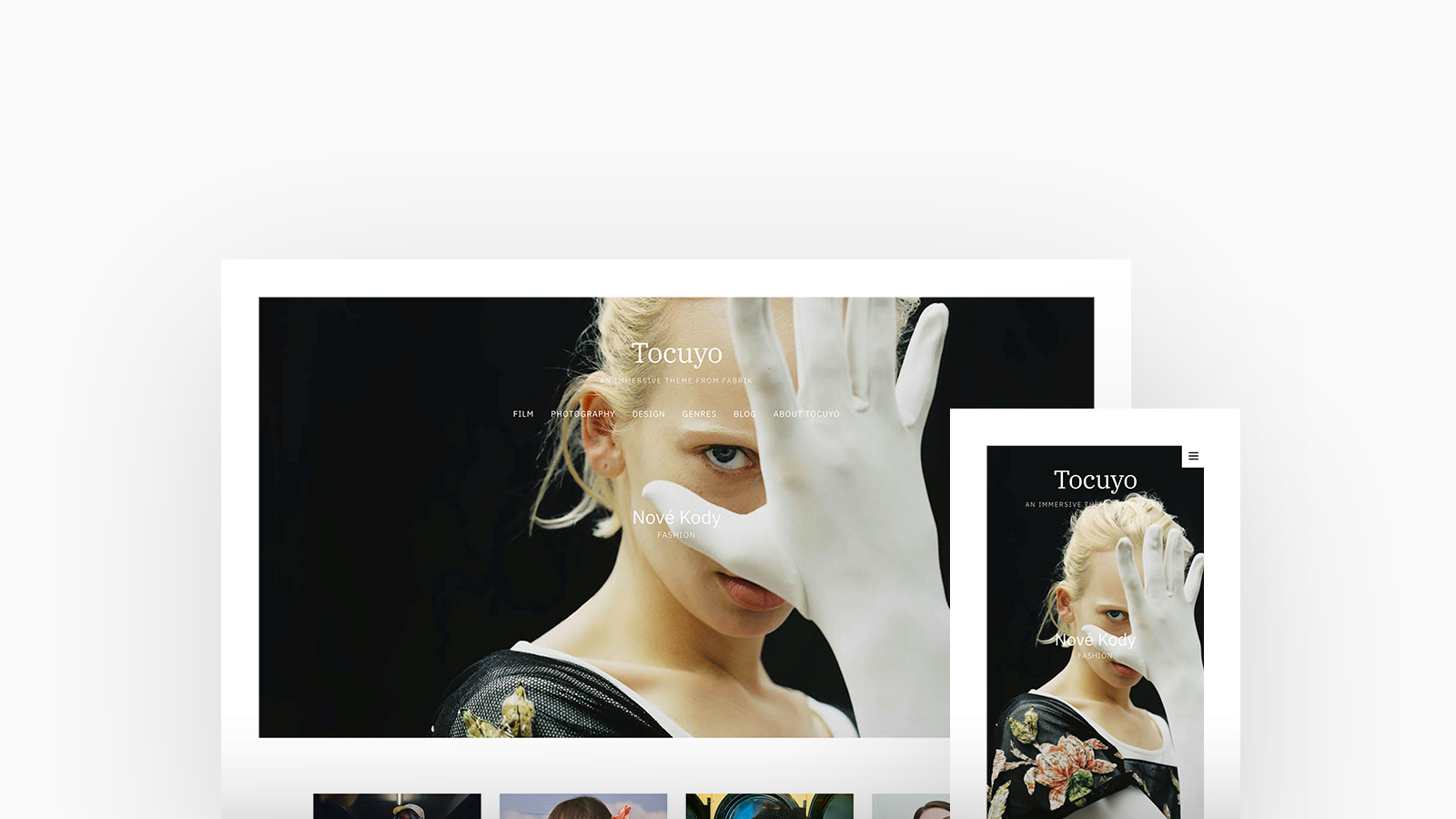The image is a layered composition featuring a young woman with blonde hair pulled back, some strands falling over her ears. She has striking blue eyes and wears a black dress adorned with pink floral patterns. Her right hand, clad in a delicate white glove, is positioned in front of her face, with her thumb and forefinger encircling her eye, partially covering her lips which form a closed, serene expression.

There are two versions of the same photo in the image: one in a horizontal layout stretching from left to right, and the other in a vertical layout positioned at the bottom right corner. Both photos are bordered by a white frame and have the word "Tocuyo" written in white letters, either across her forehead or to the side. The background within each frame is black, enhancing the contrast and focus on the young woman.

Each element of the composition, from the repetition of the image to the framing and text, adds to the overall intricate presentation of the photograph.